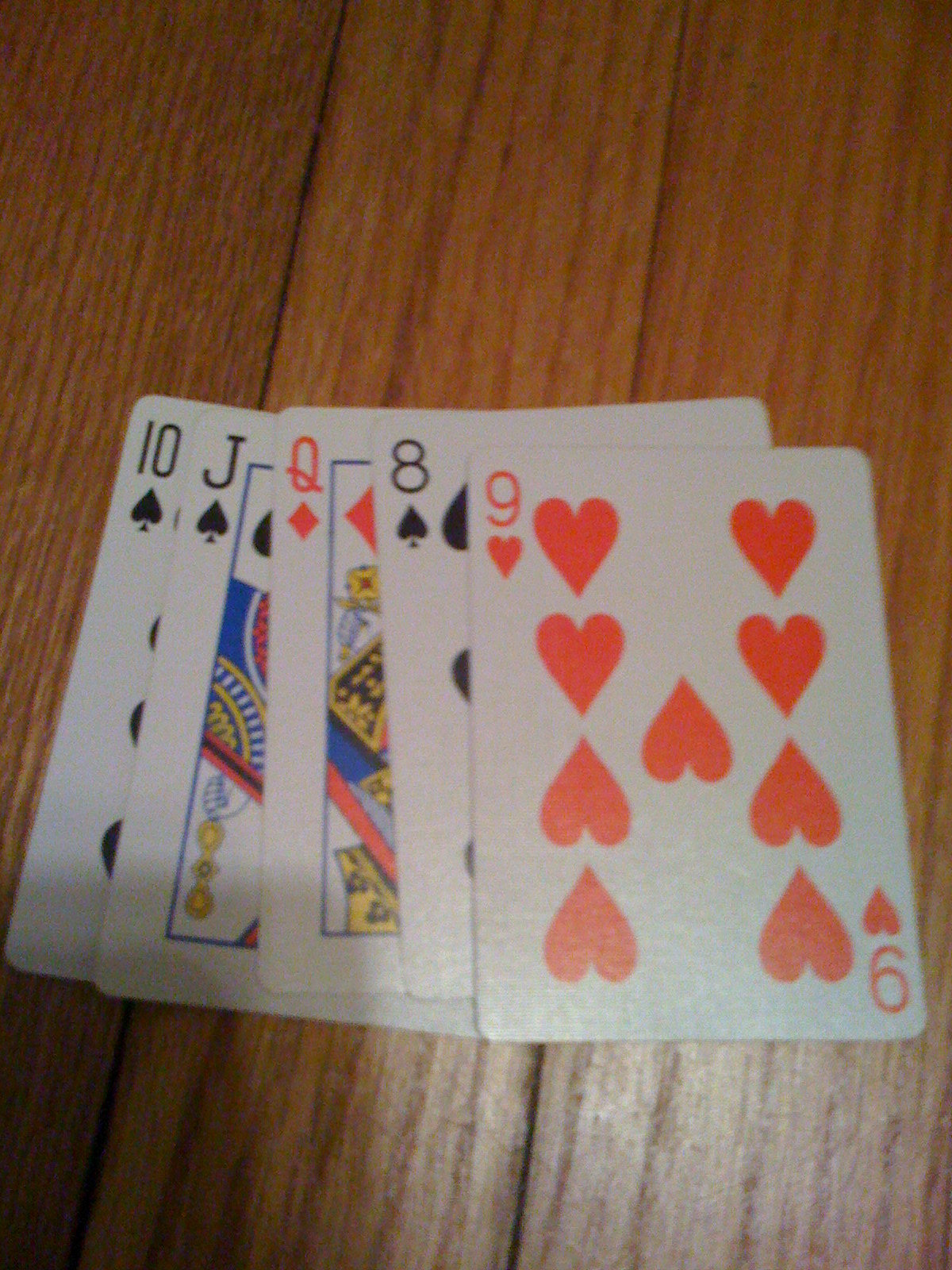In this close-up, rectangular photograph with a portrait orientation, a stack of face-up playing cards is meticulously arranged atop a medium brown wooden table featuring vertical grains. The visible part of the stack showcases an array of cards in a specific sequence: the 10 of spades, the jack of spades, the queen of diamonds, the 8 of spades, and the 9 of hearts. The 9 of hearts, positioned at the top, is fully visible and prominently displays its design. The card has a large red heart under the number nine at the top, followed by two rows of four hearts each—two upright hearts in the top row and two upside-down hearts in the bottom row, with an additional solitary upside-down heart at the center. The composition highlights the intricate details of the playing cards against the natural wooden texture of the table.